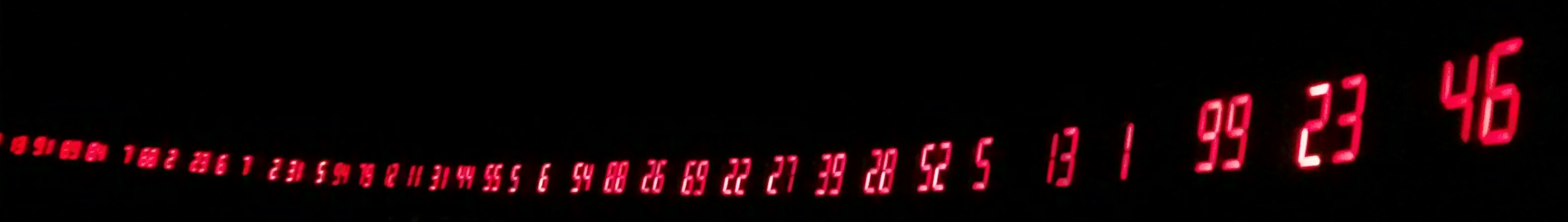The image features a long, landscape-oriented black rectangular banner, approximately 10 inches wide and 4 inches tall, showcasing a series of illuminated red digital numbers that form a subtly curved line. This curve stretches from the lower left to the upper right of the banner. The string of numbers begins small and indistinct at the lower left but grows larger and clearer as it moves rightward. Most notably, the numbers displayed are: 2, 31, 5, 12, 11, 31, 44, 55, 54, 88, 26, 69, 22, 27, 39, 28, 52, 5, 13, 1, 99, 23, and 46. These digits, rendered in an old-fashioned LED style, seem to float against the black background, evoking an impression of digital lights hanging in the night sky. Despite the clear display of numbers, the image lacks any labels or contextual details explaining its purpose or meaning.